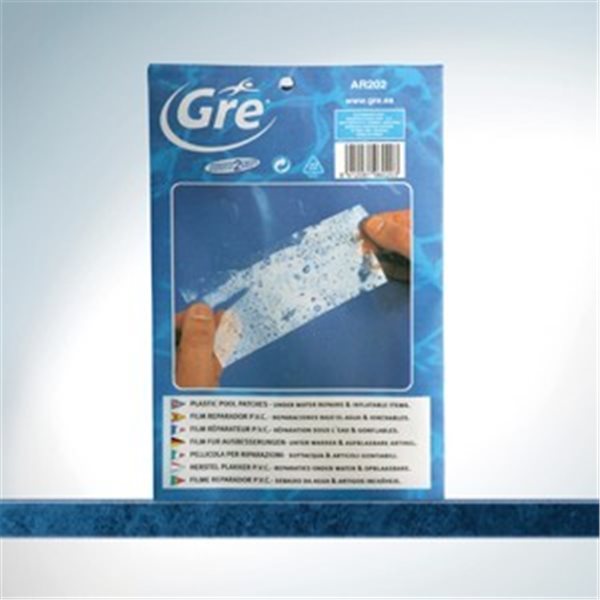This product image features a PVC repair film by the company GRE. The product is encased in blue packaging with prominent bright blue accents along the sides, top, and bottom. The top left of the package displays the word "GRE" in white letters, enclosed within an incomplete oval. Above the letter "R" is a stick figure jumping with hands raised. The package's top right corner features the string "AR202." 

The center of the packaging illustrates a person's fingers holding a thin transparent sheet with water droplets, indicating the film's water-resistant properties. The hand appears to hold the film taut, with the thumb and index finger visible from both the left and right sides of the image. The product itself rests on a blue platform symbolizing water.

The background comprises two shades of grey; the top part is darker, and the bottom and middle sections are lighter, enhancing the product's visibility. Additional details on the package include a barcode in a white rectangle in the upper right corner and small, hard-to-read text in various languages at the bottom. The overall impression is slightly unfocused, possibly due to a low-resolution image, but the key elements and branding are clear.